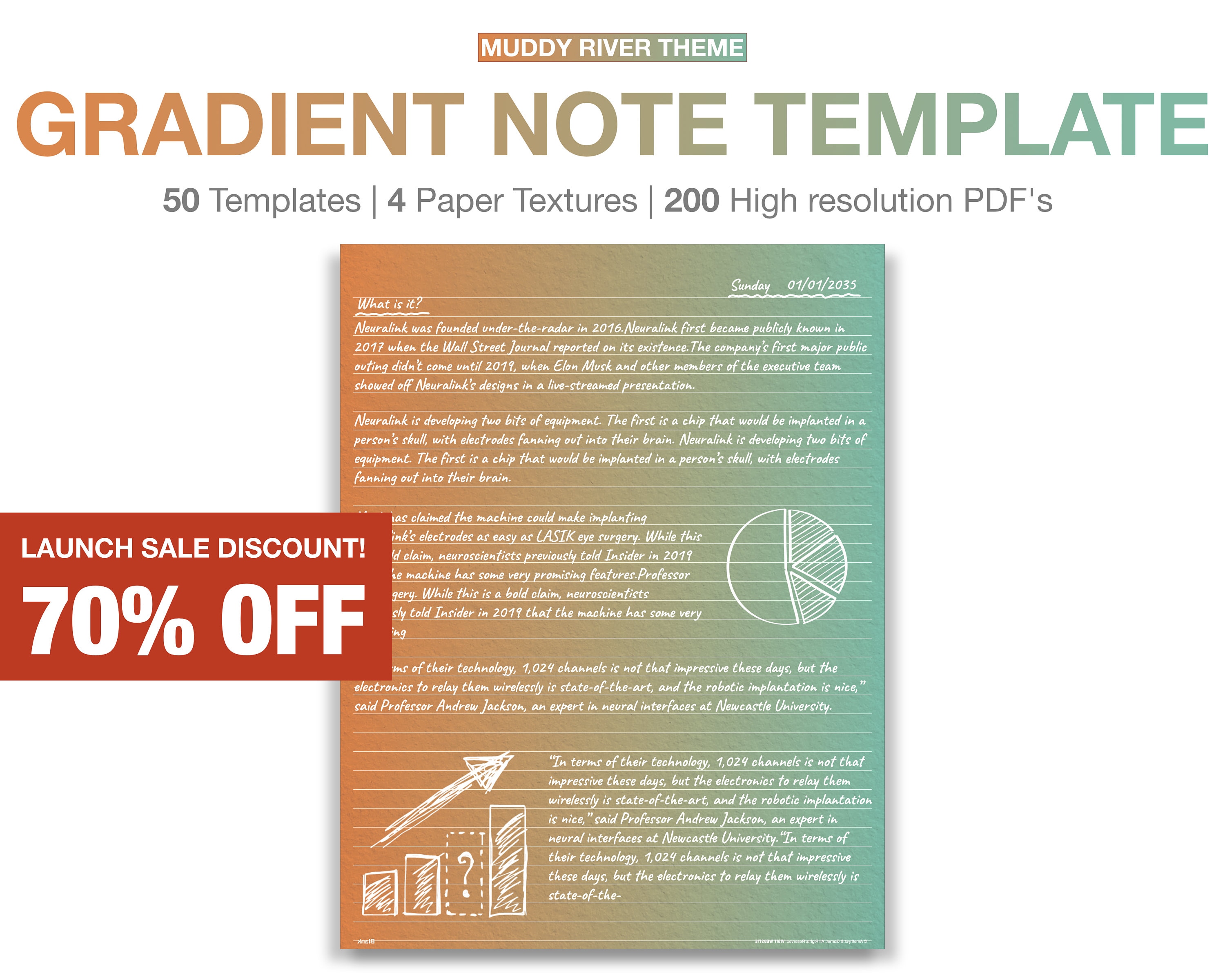This advertisement features the Muddy River Theme Gradient Note Template, prominently displayed at the top in gradient colors transitioning from peach to light blue. Beneath this title, the ad details the product's offerings: 50 unique templates, 4 distinctive paper textures, and 200 high-resolution PDFs. A red box with white text on the left announces a "Launch Sale Discount, 70% off." The main visual element is an example of the template itself, which showcases a handwritten-style font and white illustrations on a multicolored background, transitioning from brownish-peach on the left to light blue on the right. This visual is designed to demonstrate the template's distinctive aesthetic, reminiscent of chalk on a chalkboard, which sets it apart from typical digital fonts.